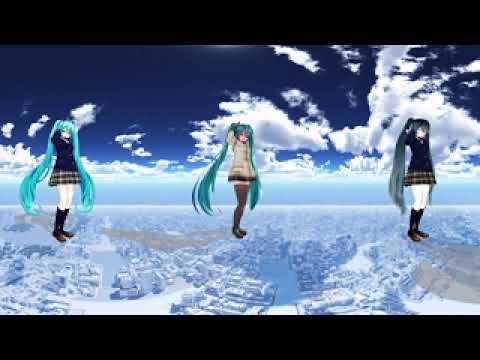In the blurred image, there are three anime-style characters resembling Hatsune Miku, floating above a snowy city with patches of clouds and a backdrop of an extraordinarily blue sky that suggests a high altitude, almost like a view from a plane. Each character has extremely long, ankle-length hair, varying in shades from a neon greenish-blue on the left, a darker bluish-green in the middle, to a grayish blue on the right. All three sport long boots; the characters on the left and right are dressed in matching schoolgirl uniforms, featuring closed blouses with ties, plaid skirts, and dark boots. The middle character distinguishes herself with a thick whitish coat and long black stockings, indicative of a winter outfit. Their floating position over the city creates a surreal scene.